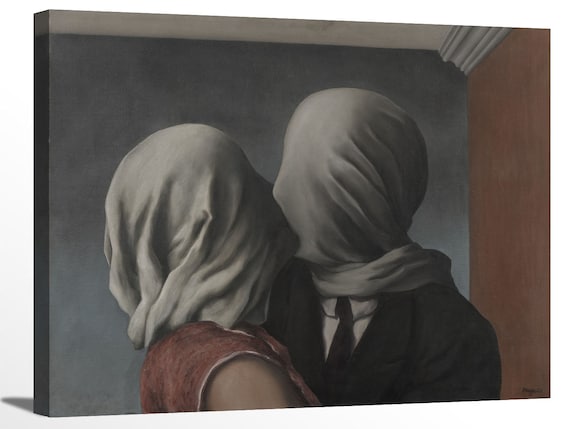This painting depicts a couple kissing while their heads are covered by white sheets, creating a poignant yet mysterious scene. The woman, positioned on the left, wears a vivid red dress, visible from a side view just above the shoulder. She faces a man on the right, who is dressed in a black suit, white shirt, and black tie. Both figures press close together, attempting to kiss through the cloth that obscures their features. The backdrop consists of a dark, grayish-blue wall with subtle light variations, contrasting with a brown wooden wall on the right that extends to a white ceiling. A trim board is visible along the brown wall, but not on the main focal wall. This setting, with its juxtaposed colors and textures, frames the tender yet enigmatic interaction between the two shrouded figures.